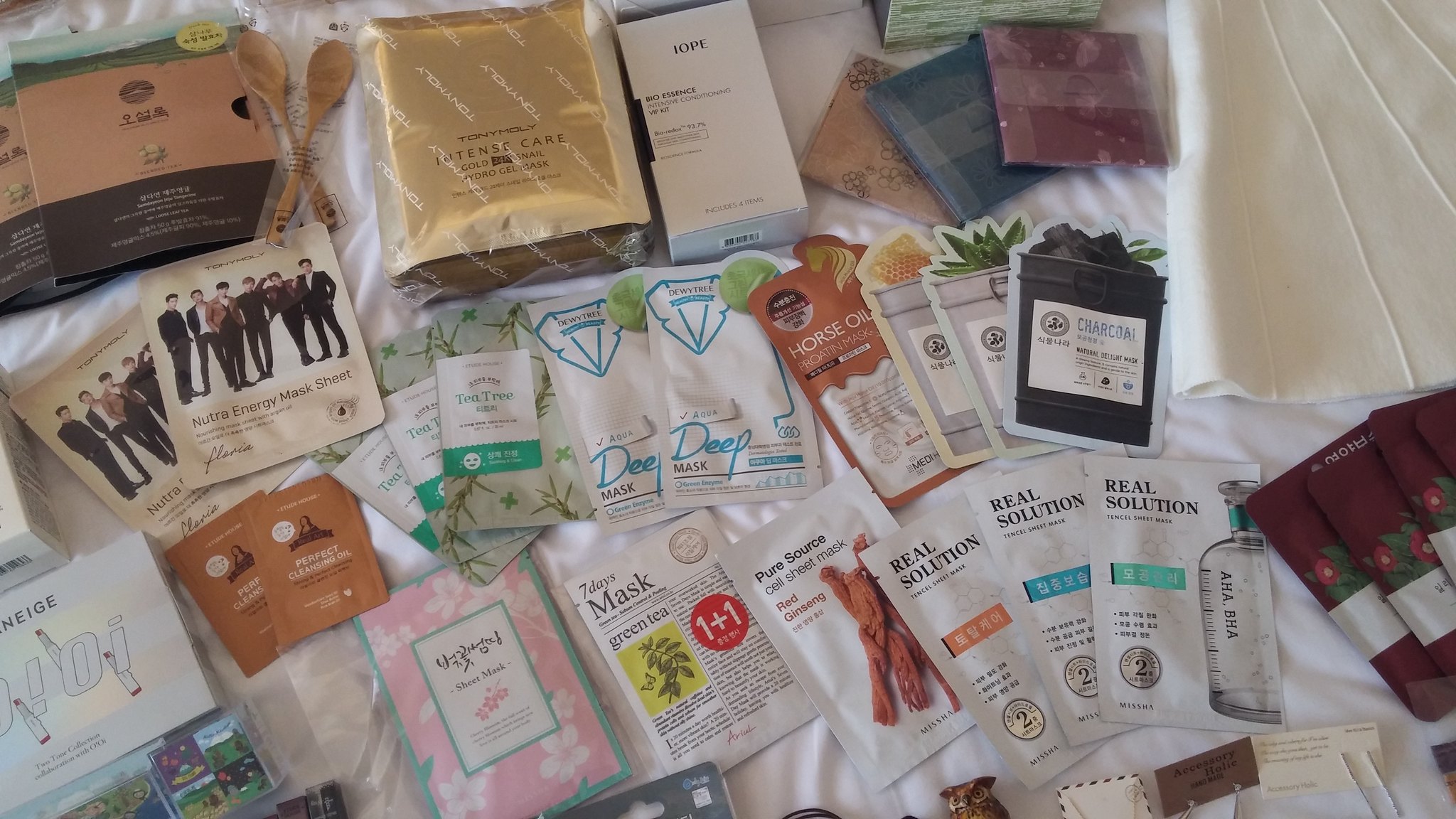The photograph showcases an array of beauty products meticulously arranged on a white sheet atop a bed. The collection primarily consists of flat-pack items such as facial and hair masks, predominantly packaged in white material featuring various logos and product information. In the top right corner, a piece of fabric, possibly a skirt, is visible, while in the bottom right corner, several maroon-colored items are present.

Noteworthy imaginative packaging can be seen among the beauty products, with some designed to resemble flower pots, complete with plant-top lids, and others decorated to look like shirts. Towards the top of the image, several bulkier box packages are present, though their exact contents are indistinct. Two of these products are adorned with images of a boy band.

Additional items in the scene include two small wooden spoons and an assortment of products extending just beyond the bottom edge of the photograph. The overall arrangement vividly portrays a diverse and creative assortment of beauty and cleaning solutions.